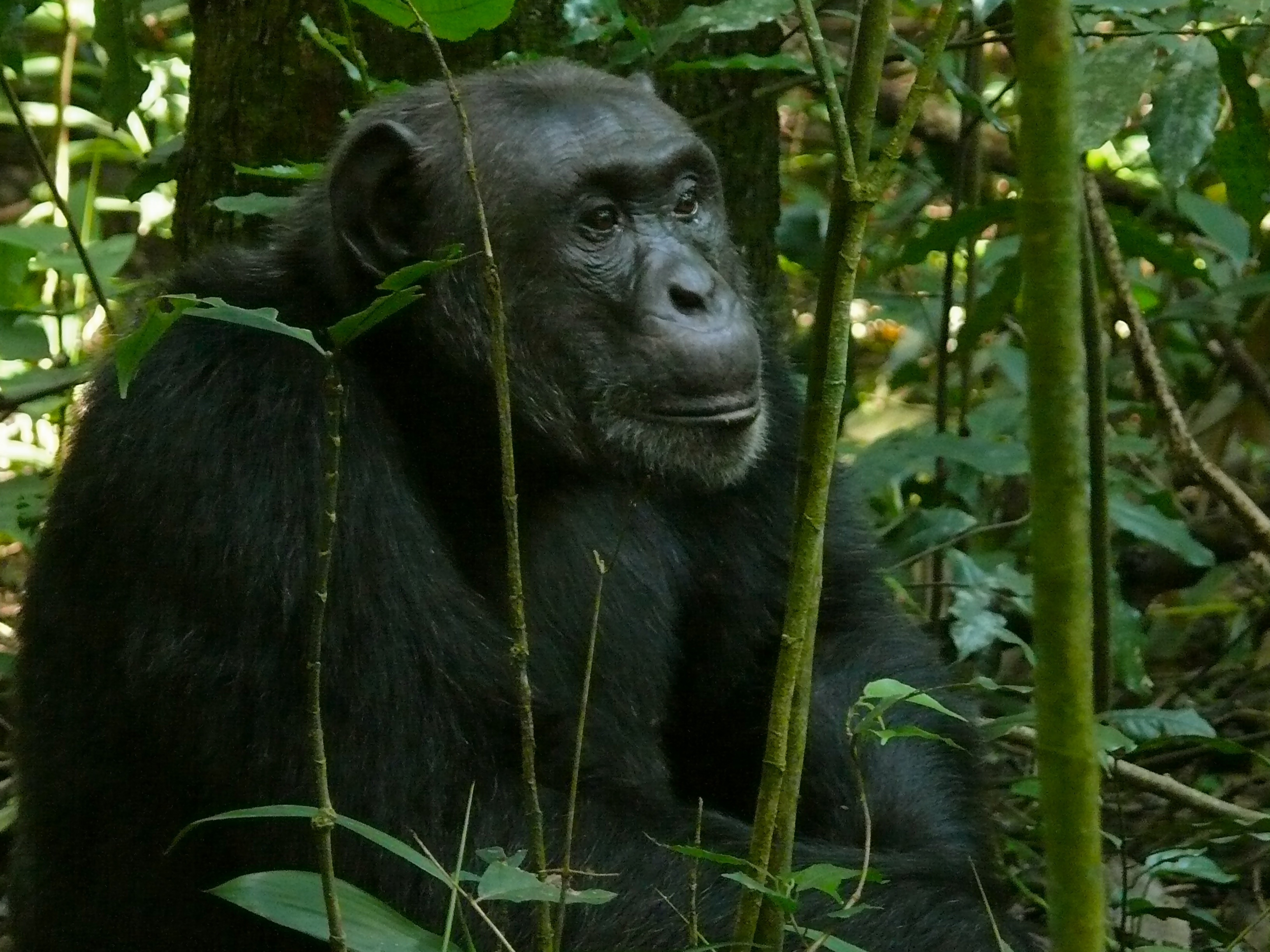The image features a black-furred ape, likely a gorilla, situated in a dense, verdant jungle filled with trees, leaves, and branches. Captured in a candid daytime photo, the ape is depicted from the midsection up and viewed in profile, facing to the right at a 45-degree angle. The scene is bathed in natural light filtering through the forest canopy, highlighting the gorilla's contemplative expression and slightly sad demeanor. Visible details include the ape's prominent ear, mouth, nose, and both eyes and arms, partially obscured by thin twigs and small branches in the foreground. The dense foliage forms a lush, green backdrop, emphasizing the jungle setting.